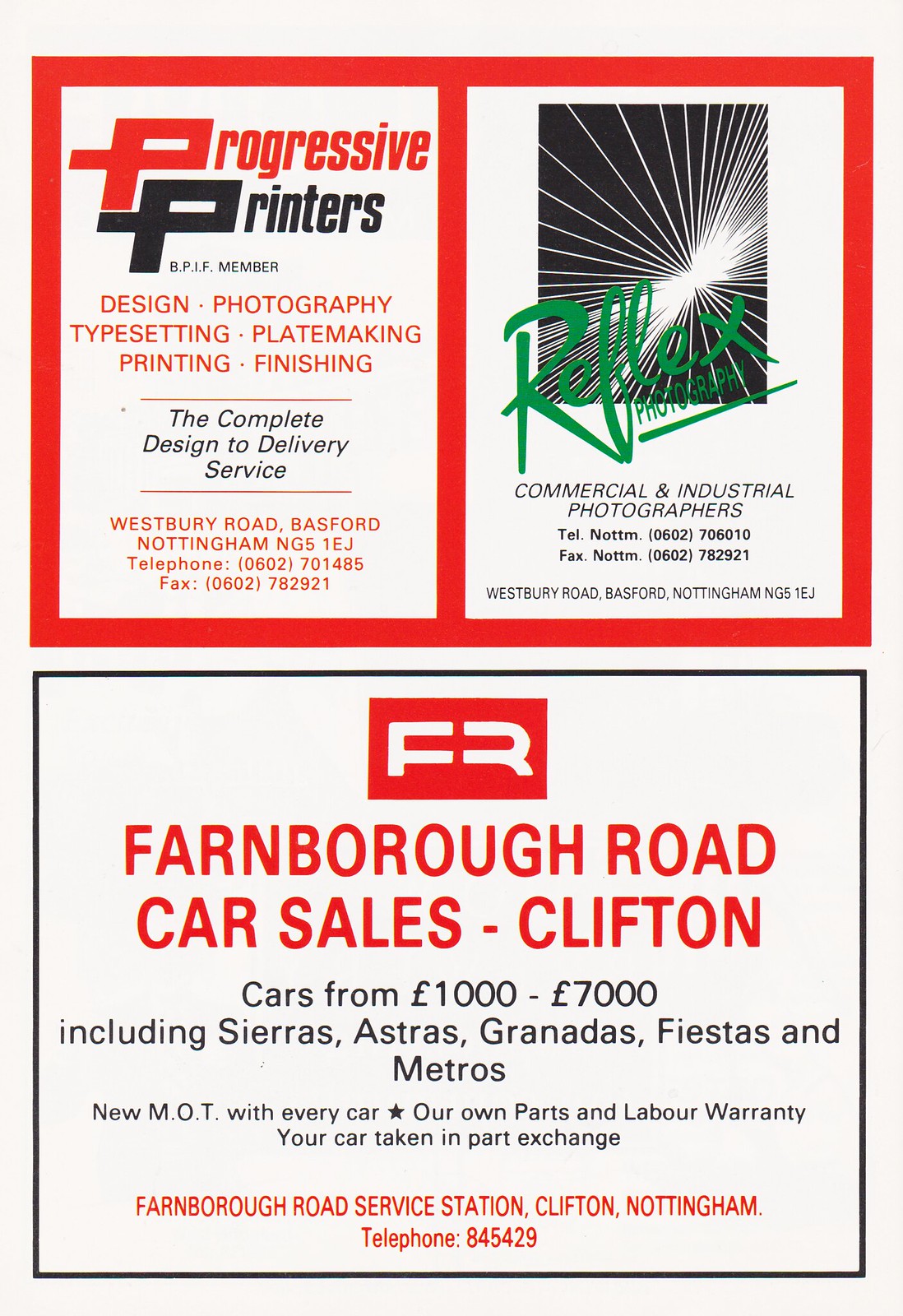The rectangular image features three distinct advertisements reminiscent of a newspaper layout, arranged in a structured, grid-like format. The top half of the rectangle consists of two equal-sized ads outlined in red borders. 

The ad on the left is for "Progressive Printers," prominently displayed in red and black text. It lists their comprehensive services in red, including design, photography, typesetting, plate making, printing, and finishing, followed by the tagline, "the complete design to delivery service." The address is noted as Westbury Road, Bassford, Nottingham, NG5, 1EJ, along with telephone and fax numbers.

To the right, the adjacent ad features a black and white starburst image overlaid with the word "Reflex" in bright green, highlighting their specialization in commercial and industrial photography. It also includes telephone numbers and the address—Westbury Road, Eastford, Nottingham.

Occupying the bottom half of the page is the larger ad for "Farnborough Road Car Sales Clifton." The logo, featuring a white 'F' and partial 'R' on a red background, sits prominently at the top. The ad offers cars ranging from £1,000 to £7,000 with mentions of various models like Sierras, Astras, Granadas, Fiestas, and Metros. Additional details include a new MOT with every car, an in-house parts and labor warranty, and the acceptance of part-exchange vehicles. The address and telephone number are also provided.

Overall, the advertisements effectively utilize color and space to convey detailed information about each business, reflecting a typical old-fashioned newspaper ad layout.